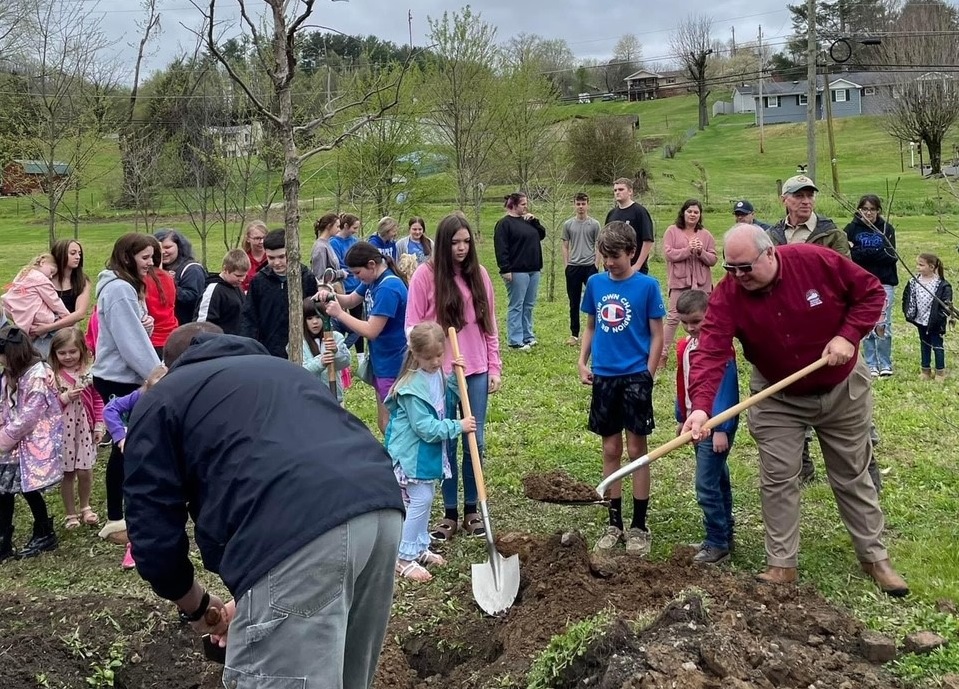This photograph captures a lively community event where a group of over 20 people, comprising both adults and children, are actively engaged in digging or filling a large hole in a grassy field. Central to the scene is an older man with a balding head, wearing a red collared shirt and brown pants, energetically using a shovel to move dirt. Nearby, a young girl dressed in a blue jacket and jeans also busies herself with a shovel, symbolizing the enthusiastic involvement of the younger generation in the activity. Surrounding these key figures are numerous other participants, predominantly children, eagerly helping with shovels as well. The scene is set against a backdrop of green grass, small trees, and at least six houses dotting a hillside. The sky is overcast, adding a gray hue to the otherwise vivid and bustling environment marked by its sense of communal effort, perhaps linked to a tree-planting initiative or Earth Day celebration.